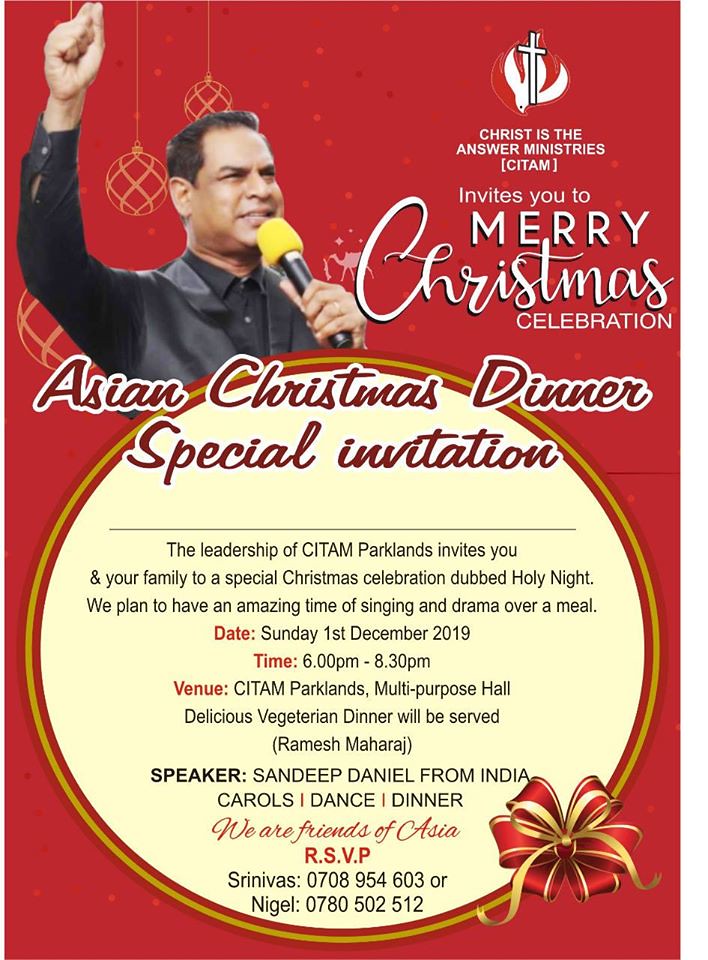The image is a color advertisement for a special Christmas event hosted by Christ is the Answer Ministries (CITAM). It features a head-and-shoulders cutout of a man with dark hair and skin, dressed in a black vest over a black shirt, holding a yellow microphone. The text is primarily red and includes a stylish "Merry Christmas" greeting and an "Asian Christmas Dinner Special Invitation." The leadership of CITAM Parklands invites you and your family to a special Christmas celebration dubbed "Holy Night," featuring an evening of singing, drama, and a delicious vegetarian dinner. The event takes place on Sunday, December 1st, 2019, from 6 p.m. to 8:30 p.m. at the CITAM Parklands Multipurpose Hall. The featured speaker is Sandeep Daniel from India. Carols, dance, and dinner will be part of the program. For RSVPs, contact Srinivas at 0708-954-603 or Nigel at 0780-502-512. At the bottom right, there is a tied golden-red Christmas bow, adding a festive touch.